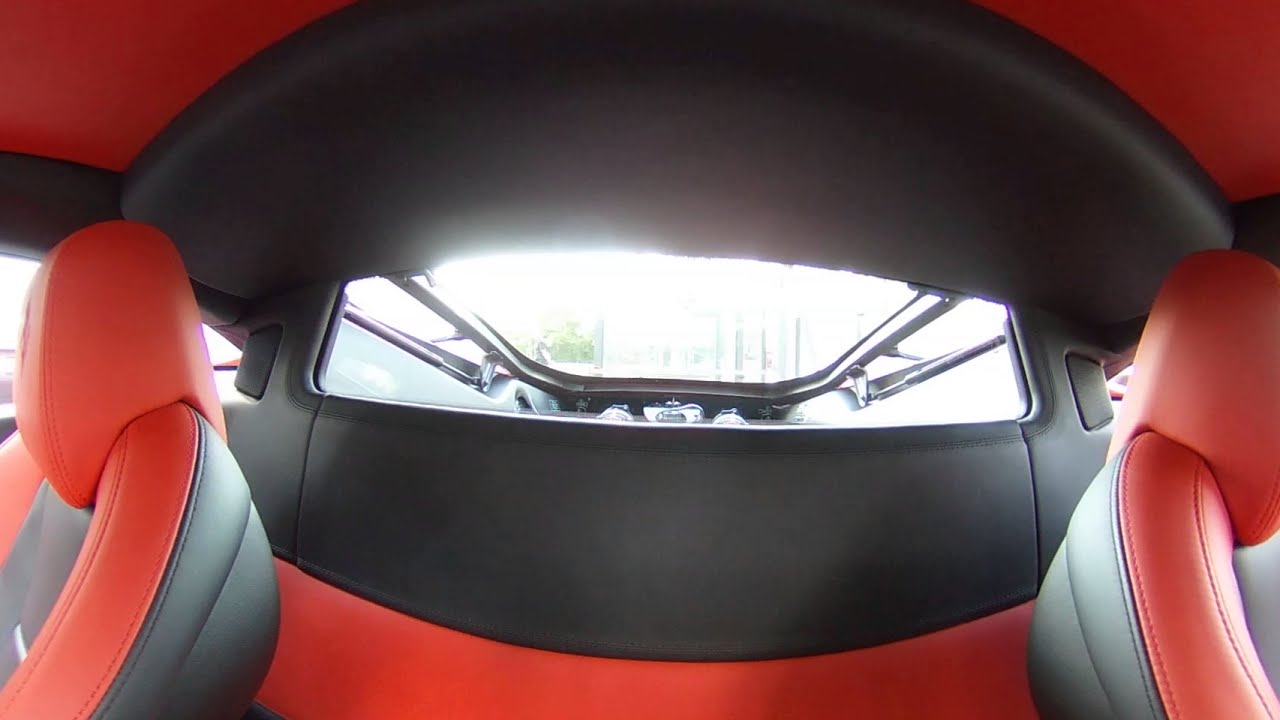The image captures the interior of a unique sports car, viewed from the back towards the rear windshield. The car features a striking black and red color scheme, with cushions and most of the interior upholstered in these bold hues. The sloped rear windshield, held by hydraulic arms, sheds light on the scene with sunlight pouring in, offering a view of the engine just beneath it. The ceiling is mostly black, and the car is equipped with speakers on each side. Outside the rear windshield, one can see a person in a black shirt walking on the street. Additionally, there are several cars parked nearby and buildings with green trees in the distance. The scene is bathed in daytime sunlight, illuminating the rich details inside and outside the vehicle.